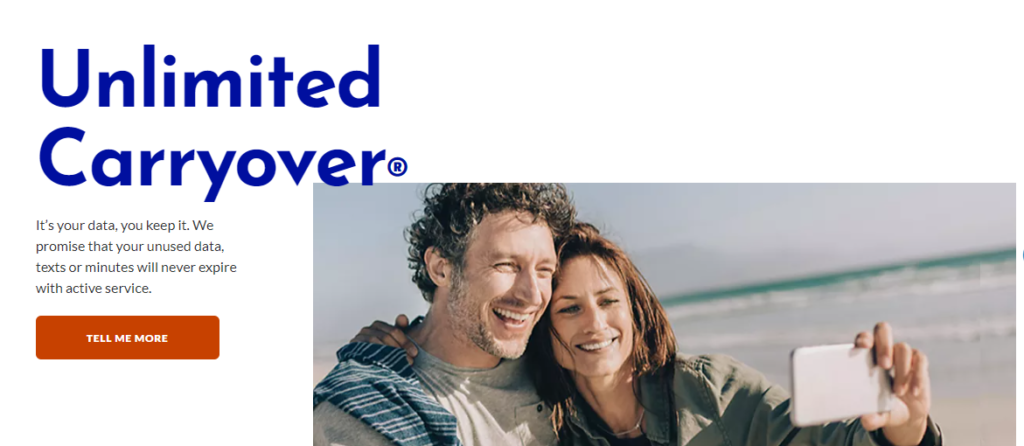This image is a screenshot from a website with a clean, white background. At the top left, there is a prominent headline: "Unlimited Carryover" with "Unlimited" on the top line and "Carryover" right beneath it. Accompanying the text, there is a small circular icon with a capital 'R' inside, rendered in dark blue. Below this, the text explains the feature: "It's your data. You keep it. You promise that your unused data, texts, or minutes will never expire with active service."

Further down, an orange-red rectangular button with white, all-capital letters reads "TELL ME MORE," inviting users to click for additional information. To the right of this text section, an outdoor image is displayed. The background features a blue-gray sky with thick, puffy white clouds. Below the sky, the scene captures the ocean with waters depicted in a greenish hue, transitioning to white waves cresting towards the shore, which meets the sand.

In the foreground, a man and a woman appear from the upper chest up, standing side by side with their heads close together. The woman, slightly shorter than the man, extends her arm holding a cell phone, capturing a selfie of the two against the scenic backdrop.